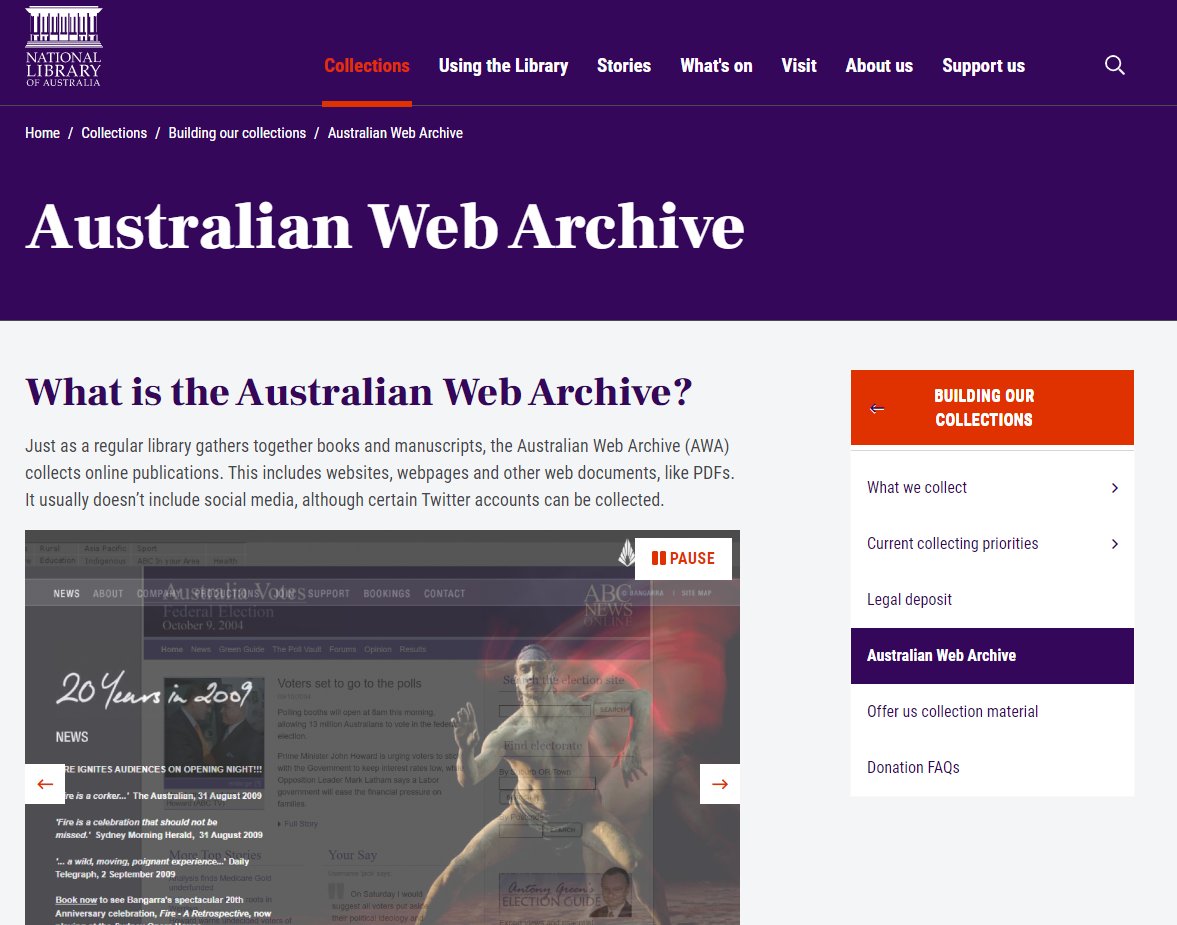The image displays the homepage of the National Library of Australia's Web Archive, specifically highlighting the Australian Web Archive (AWA). The AWA serves as a digital repository for online publications, much like a traditional library preserves books and manuscripts. It collects a diverse range of web content, including websites, webpages, and documents such as PDFs, although social media content is generally excluded, with some exceptions for selective Twitter accounts.

Prominently featured in the image is an emblem of a statue commemorating "20 years in 2009," alongside the latest news headlines. A sidebar section labeled "Building Our Collection" outlines the scope of the archive's efforts with subcategories such as "What We Collect," "Current Collecting Priorities," "Legal Deposit," and guidelines for contributing materials through "Offer Us Collection Material" and "Donation FAQs."

The page has a stylish purple background at the top, with the primary navigation menu in white text. Categories in this menu include "Collections," "Using the Library," "Stories," "What's On," "Visit," "About Us," and "Support Us." The interface also features a functional search bar for querying the archive’s holdings.

Overall, the layout effectively communicates the mission and contents of the Australian Web Archive, assisting users in navigating and understanding its extensive digital collection.